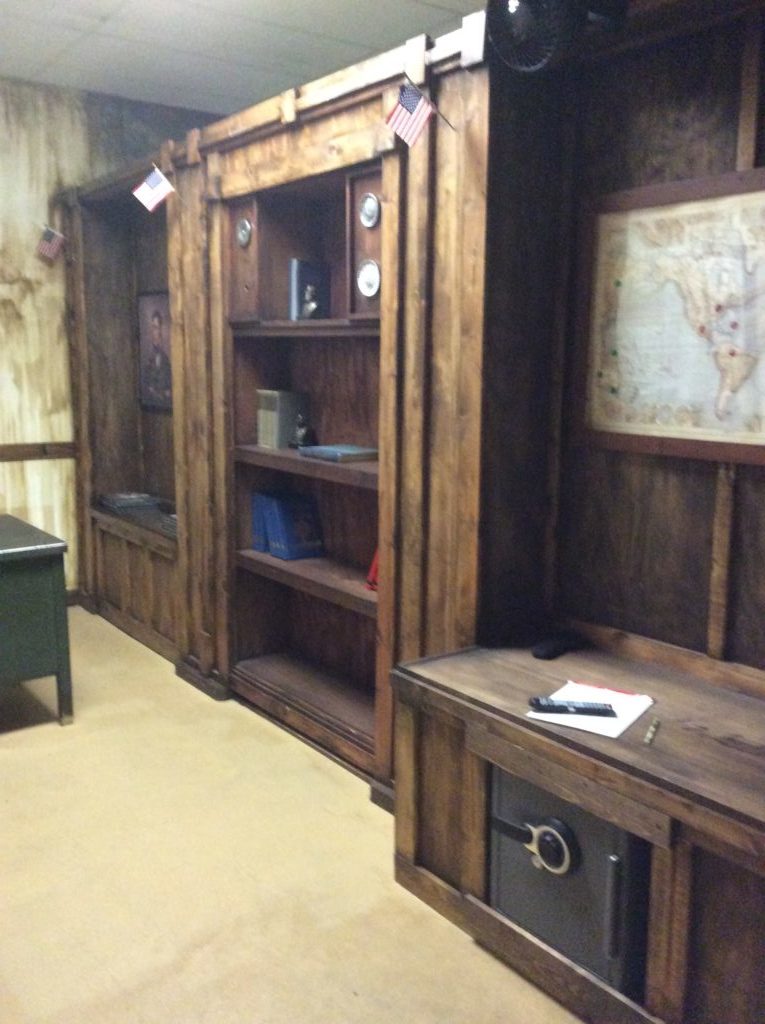This detailed color photograph, oriented in portrait, captures the interior of what appears to be a dark wood-paneled office or study area. The image showcases a three-quarter perspective of a long wall on the right, narrowing in the distance towards the left. The floor of the room is covered with tan carpet.

The central feature of the wall is an expansive wooden bookcase adorned with various items. The shelves contain a selection of books, a few framed pictures, and notably on the middle shelf, large gauge dials suggesting some sort of barometric equipment. Three small American flags are prominently placed, appearing to be affixed to the bookcase. Below the map, positioned above the chest, is a secure black safe with a turn dial. 

Directly below the map hangs a large vintage world map, further adding to the study's classic decor. This map includes red pins, possibly marking specific locations. To the left edge of the image, you can just glimpse the corner of a desk, suggesting the continuation of the room beyond the frame. Behind the desk, a tall window extends from ceiling to floor, though the view outside is not visible. This office space exudes a sense of heavy, richly textured design, punctuated by the ornate woodwork and carefully arranged items that suggest both practicality and a touch of personal character.